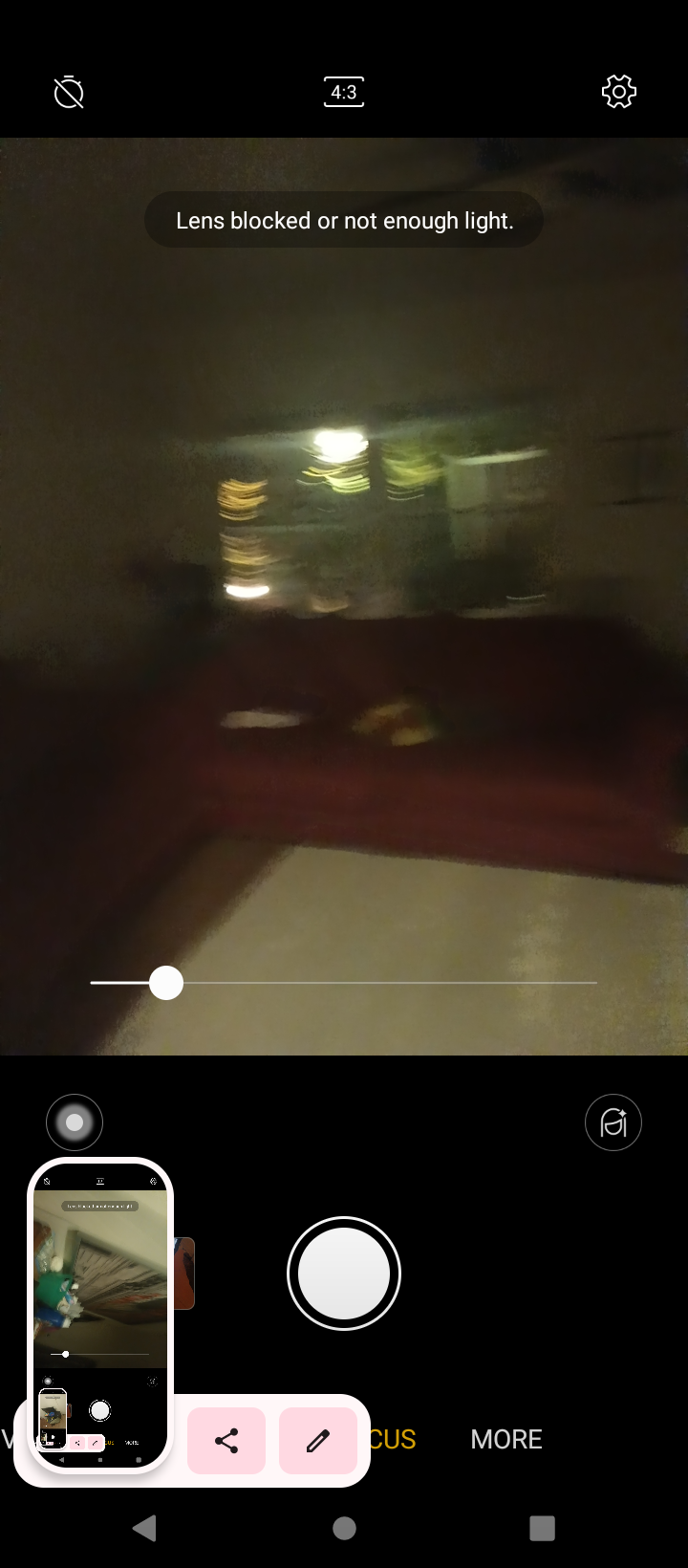This is a detailed screenshot of a phone's camera interface capturing a view of a living room. The central image in the camera app shows a red couch in a somewhat blurry background, possibly with a white tile or linoleum floor in front of it. You can faintly make out a window shape beyond the couch, with light suggesting there may be a porch outside. A notification message at the top reads "lens blocked or not enough light," indicating suboptimal conditions for taking a picture. At the top, a black bar displays the 4:3 aspect ratio and a gear icon in the red corner for settings, while the bottom of the screen features a large white button for capturing the photo. There is an inset image in the lower-left corner that shows the actual photograph area. The floor beneath the couch is white tile, and there’s a possibility of a rug nearby, adding to the domestic scene.